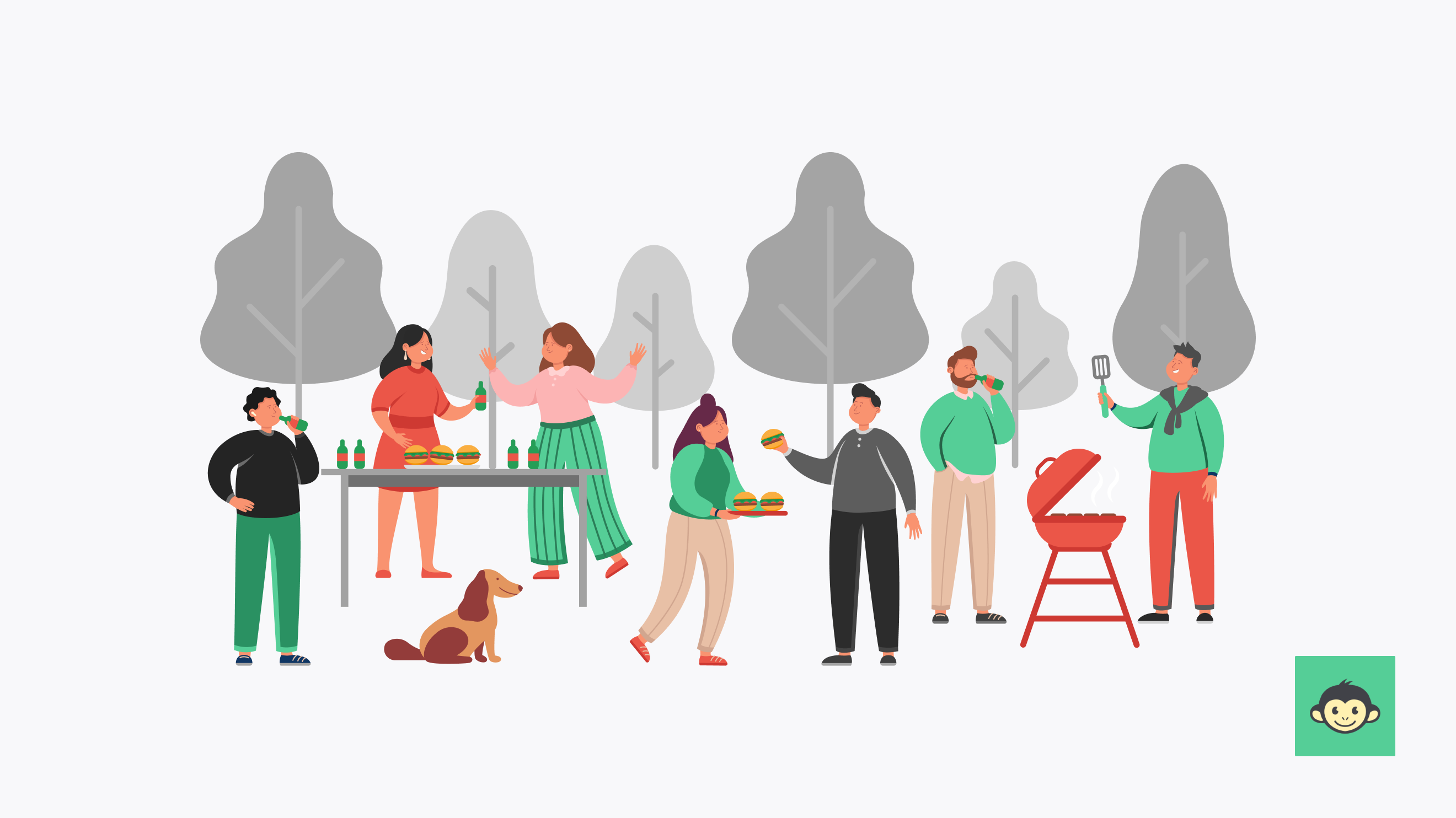In this stylized cartoon drawing set against a gray background, a group of seven people is depicted attending a barbecue in a park with six simple, monochromatic trees in the background. The scene centers around a lively gathering with a variety of interactions and details. 

From right to left, the image showcases a man in a green shirt and red pants manning the grill, energetically holding up a spatula. Next to him stands a man in green and gray attire, enjoying a beer. Beside them, a woman with long brown hair and a green shirt, contrasted with darker green sleeves and torso, is holding a plate of burgers, from which a man dressed in black pants and a gray shirt is grabbing one. Over to the left, a table set with four beers and three burgers serves as the focal point for two women conversing animatedly. One woman, sporting a pink shirt with a white collar and long brown hair, stands next to a woman in a red dress with smiling hair, gesturing with her hands. Also on the left, a solitary man dressed in a black shirt and green pants, sips on a beer. A small, happy brown dog sits contentedly beneath the table. In the lower right-hand corner, the image is subtly branded with a cartoon monkey logo set against a green background.